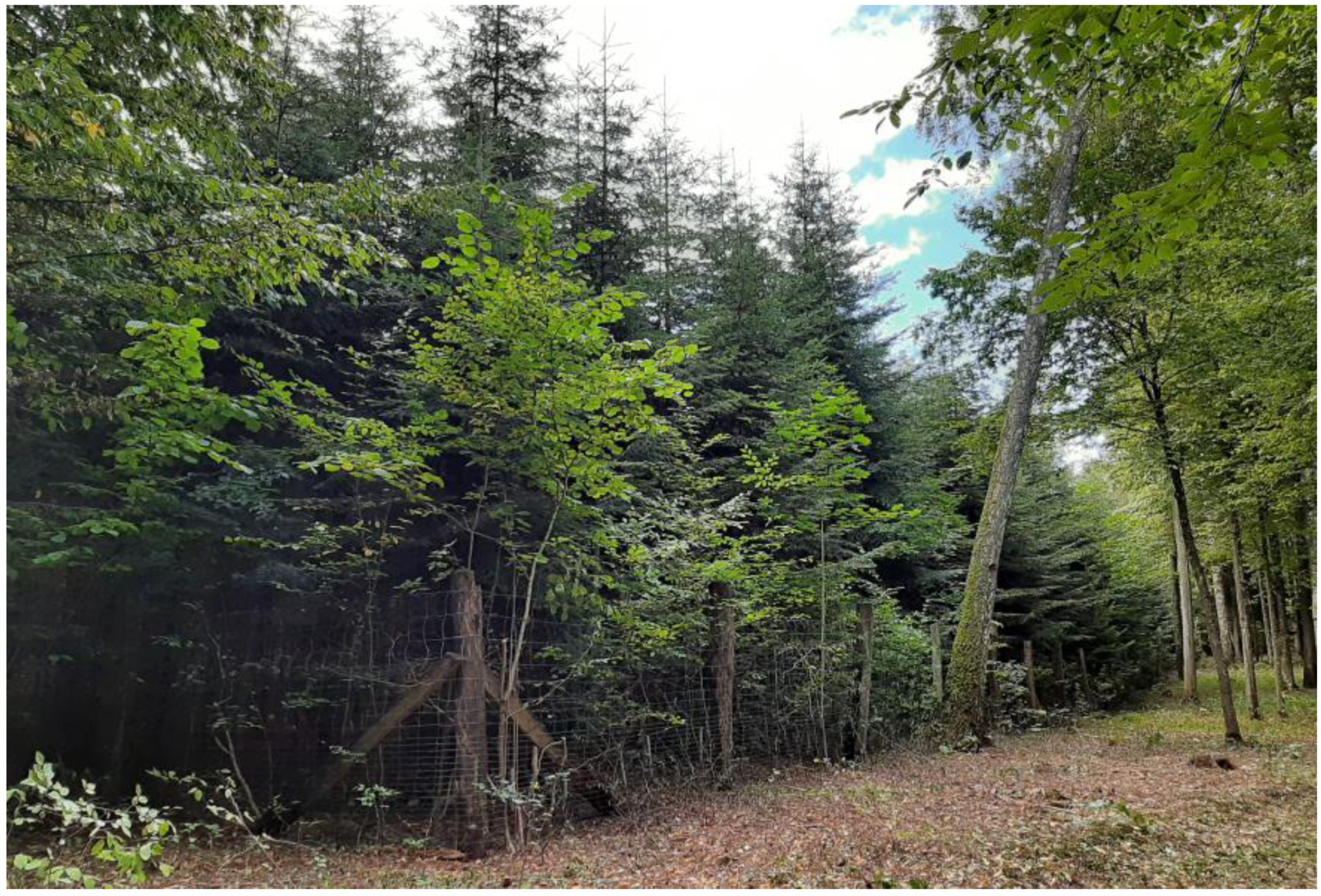The image depicts a serene forest scene featuring a dense thicket of trees, both deciduous and possibly pine or Douglas fir, adorned with green leaves and needles. The forest floor is layered with brown fallen leaves and scattered grass patches further in the distance. A prominent wooden fence bisects the image, composed of rustic tree stumps serving as fence posts, interconnected by wire fencing. The fence posts, embellished with climbing vines and plant matter, edge off into the distance, suggesting an enclosed area. At the corner of the fence, two wooden cross beams provide additional stability. To the right of this structure, a tall, leafless tree leans significantly to the right, propped by a smaller tree with green leaves, creating an intricate natural interplay. The sky above is a bright blue with a scattering of clouds, and it appears to be morning, hinted by the soft lighting. The bottom left corner of the image features a mix of leaves, sticks, and sparse ivy, adding to the rich, textured undergrowth of the forest floor.